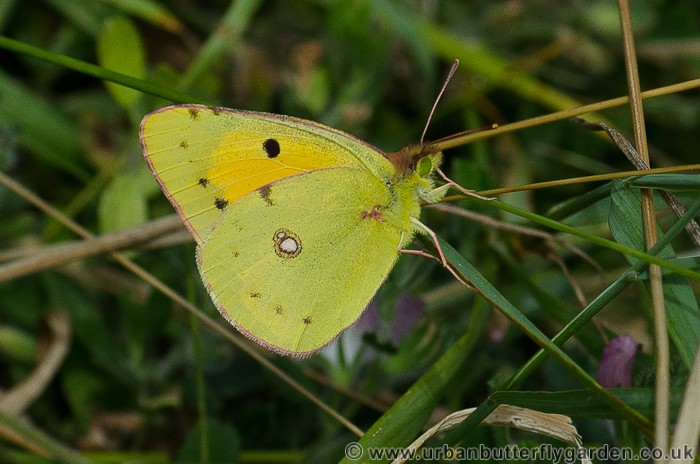This stunning close-up photograph features a yellow butterfly delicately perched on a blade of green grass, amid a grassy area adorned with a mixture of green and brown hues. Captured with a macro lens, the image showcases an intricate level of detail, from the slender, twig-like brown legs of the butterfly to its fuzzy head and emerald green eyes. The butterfly’s partially open wings, which are primarily yellow, display a unique pattern: a prominent white spot in the center, several black spots near the top, and a subtle mixture of brown and lime green shades. Equally noteworthy are the tiny purple flowers peeking through the grass in the background, adding a dash of color to the scene while the butterfly rests and nibbles on the foliage. The blurred greenery in the background enhances the focus on the butterfly, drawing the observer’s eye to its delicate features. A watermark at the bottom reads "www.urbanbutterflygarden.co.uk," subtly affirming the professional quality of the photograph.